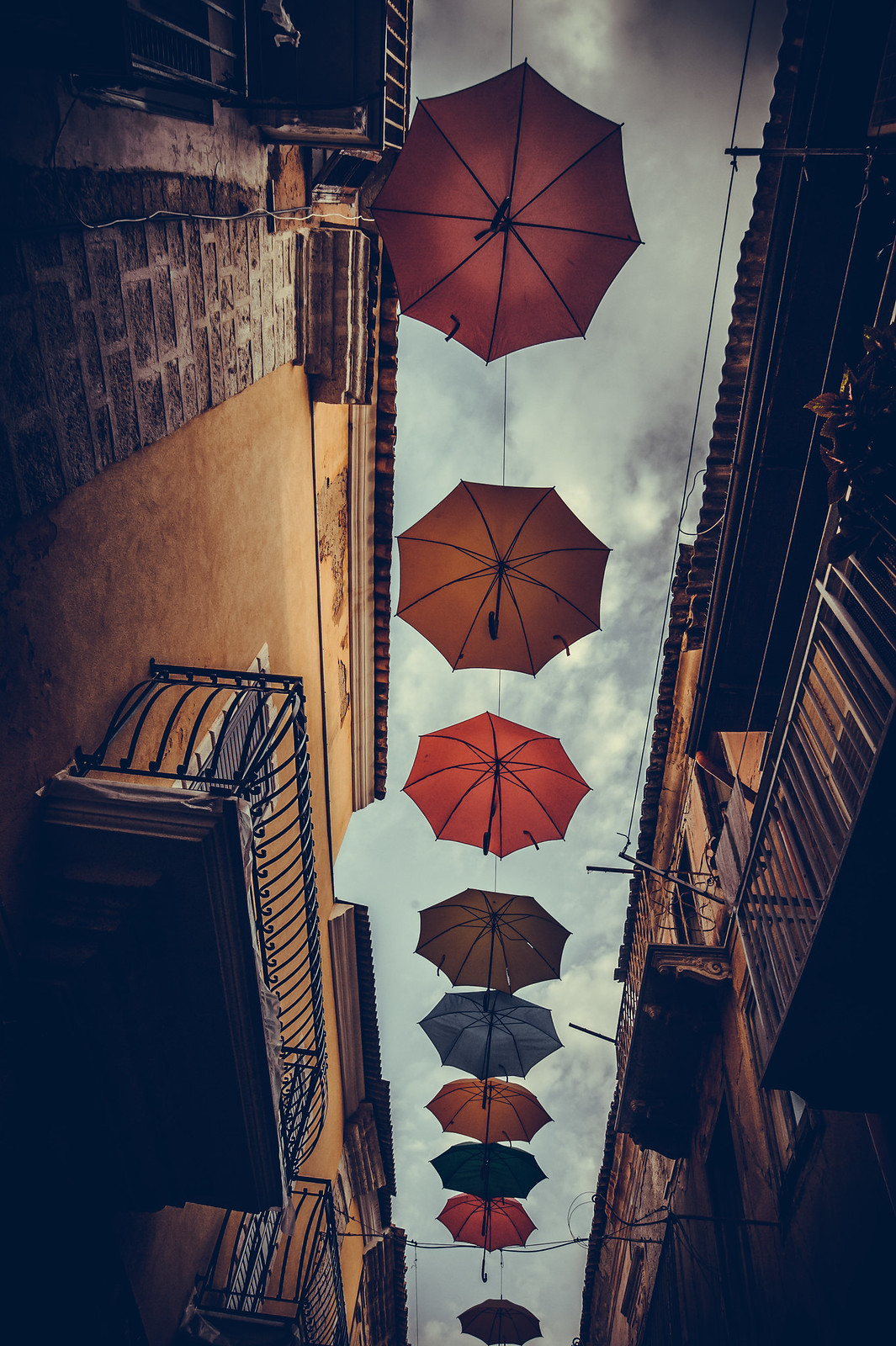This photograph, taken from the ground looking up, captures an alleyway between two old apartment buildings. The buildings, which display a mix of yellow stucco and orange brick, have ornate balconies with iron railings. In the narrow strip of sky between them, a wire stretches across, supporting a series of open, multicolored umbrellas. These umbrellas, featuring hues of brown, orange, blue, red, gray, and black, hang suspended above, adding a whimsical touch to the scene. The sky is a mix of light blue and cloudy, hinting at an overcast day. The image, possibly taken in a European or South American city, has a dark, muted filter that further emphasizes the age and character of the setting.